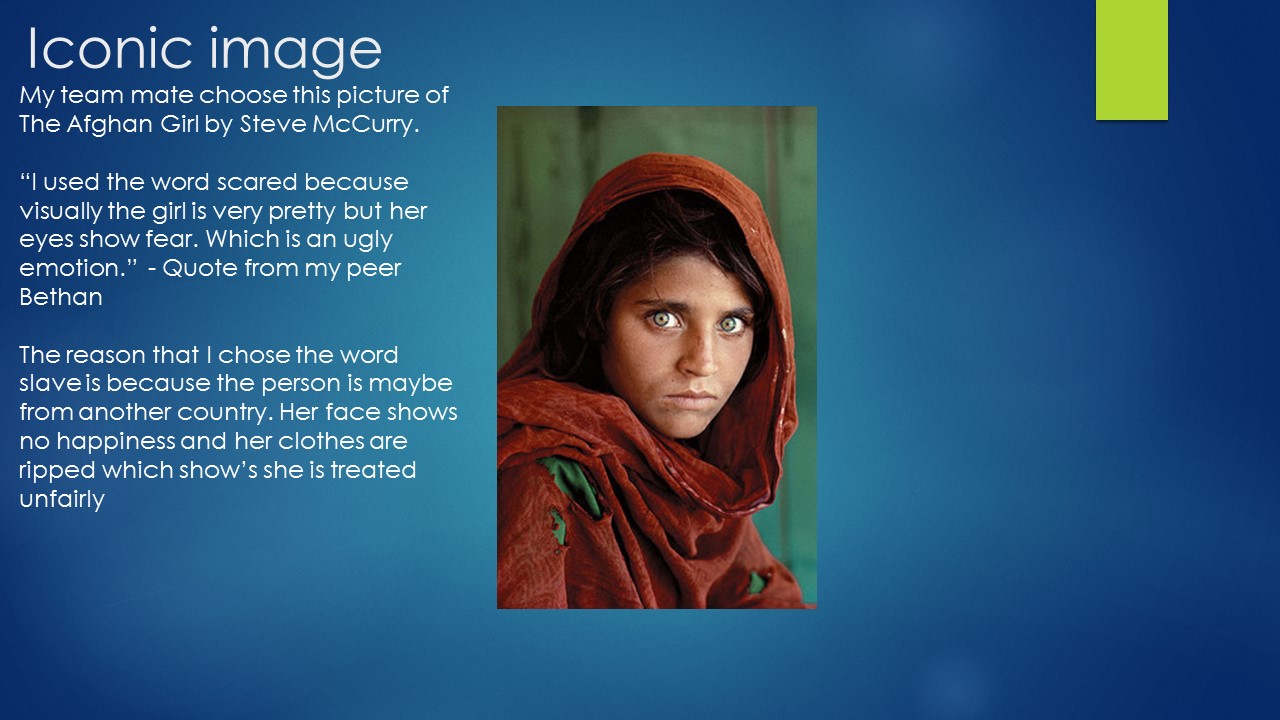The central image in this detailed, color photograph, presented as an informational slide, is the iconic portrait of the Afghan girl by Steve McCurry. This renowned photograph captures a young girl with striking green eyes, wearing a red veil and scarf, and gazing intensely at the viewer with a mix of fear and sadness. Her dark hair peeks out from the red headscarf, and her torn clothing suggests hardship and unfair treatment. The background of the slide is variegated blue, with a light green rectangle in the top right corner, containing a smaller black and pea-green square. On the left side of the image, large white text reads, "Iconic Image," followed by three paragraphs in white text. The first paragraph states, "My teammate chose this picture of the Afghan girl by Steve McCurry." The second paragraph is a quote from Bethann: "I used the word scared because visually the girl is very pretty, but her eyes show fear, which is an ugly emotion." The third paragraph expands further, explaining the choice of the word "slave" due to the girl's appearance, suggesting she is from another country and treated unfairly. This slide expertly combines photographic realism with graphic design elements to emphasize the emotional impact and historical significance of the image.